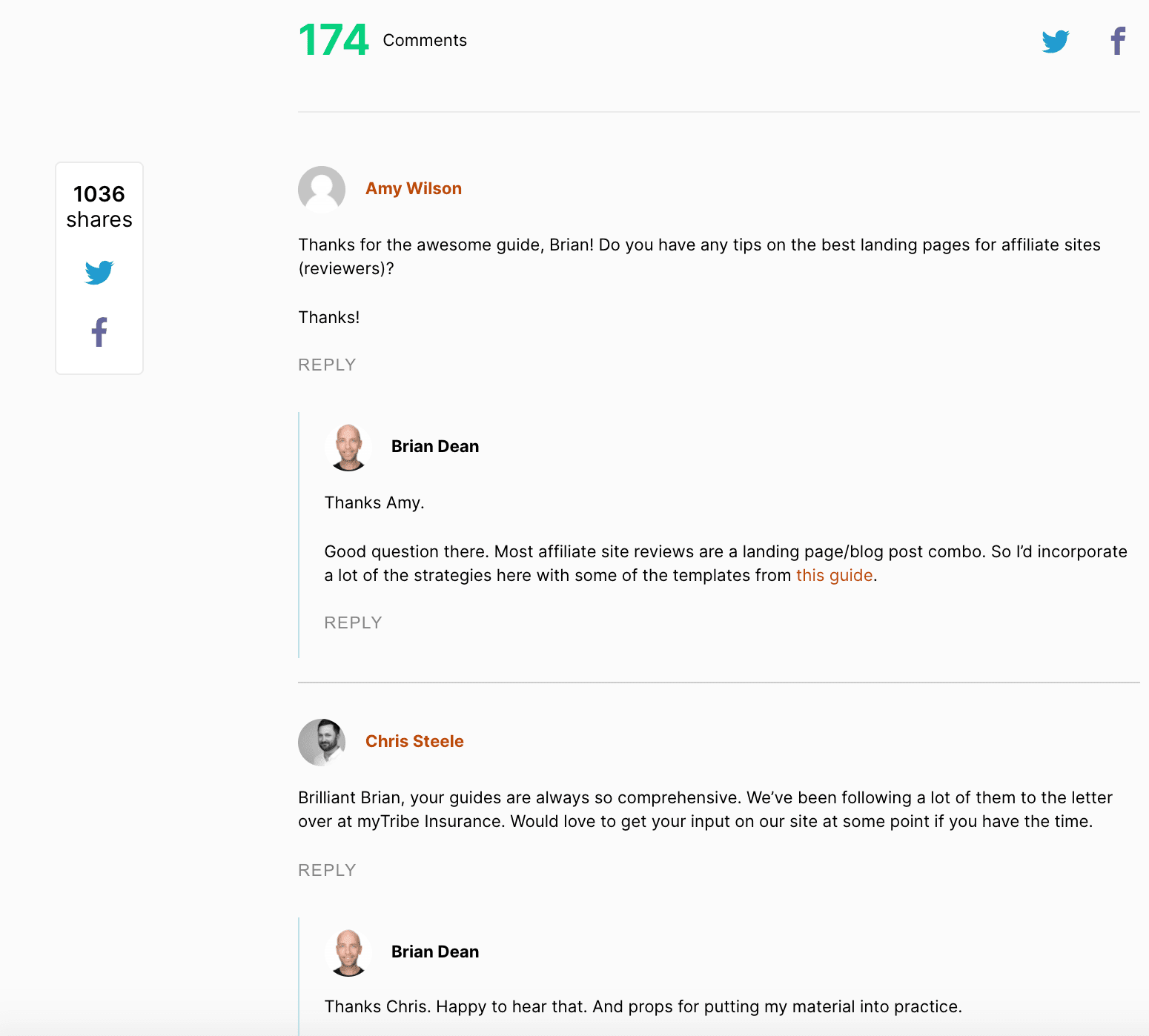The image depicts a social media exchange, likely cross-posted between Twitter and Facebook. The page has a predominantly black-and-white color scheme. At the top, a user named Amy Wilson writes, "Thanks for the awesome guide, Brian. Do you have any tips on the best landing pages for affiliate sites? Thanks." Brian Dean responds with, "Good question there. Most affiliate site reviews are landing page/blog post combos. So, I'd incorporate a lot of the strategies here with some of the templates from this guide.” Chris Steele then chimes in, "Brilliant, Brian. Your guides are always so comprehensive. We've been following a lot of them to the letter over at My Tribe Insurance. Would love to get your input on our site at some point if you have the time." Brian replies, "Thanks, Chris. Happy to hear that. And props for putting my material into practice." The page at the top indicates there are 174 comments and, to the left, it shows 1,036 shares.